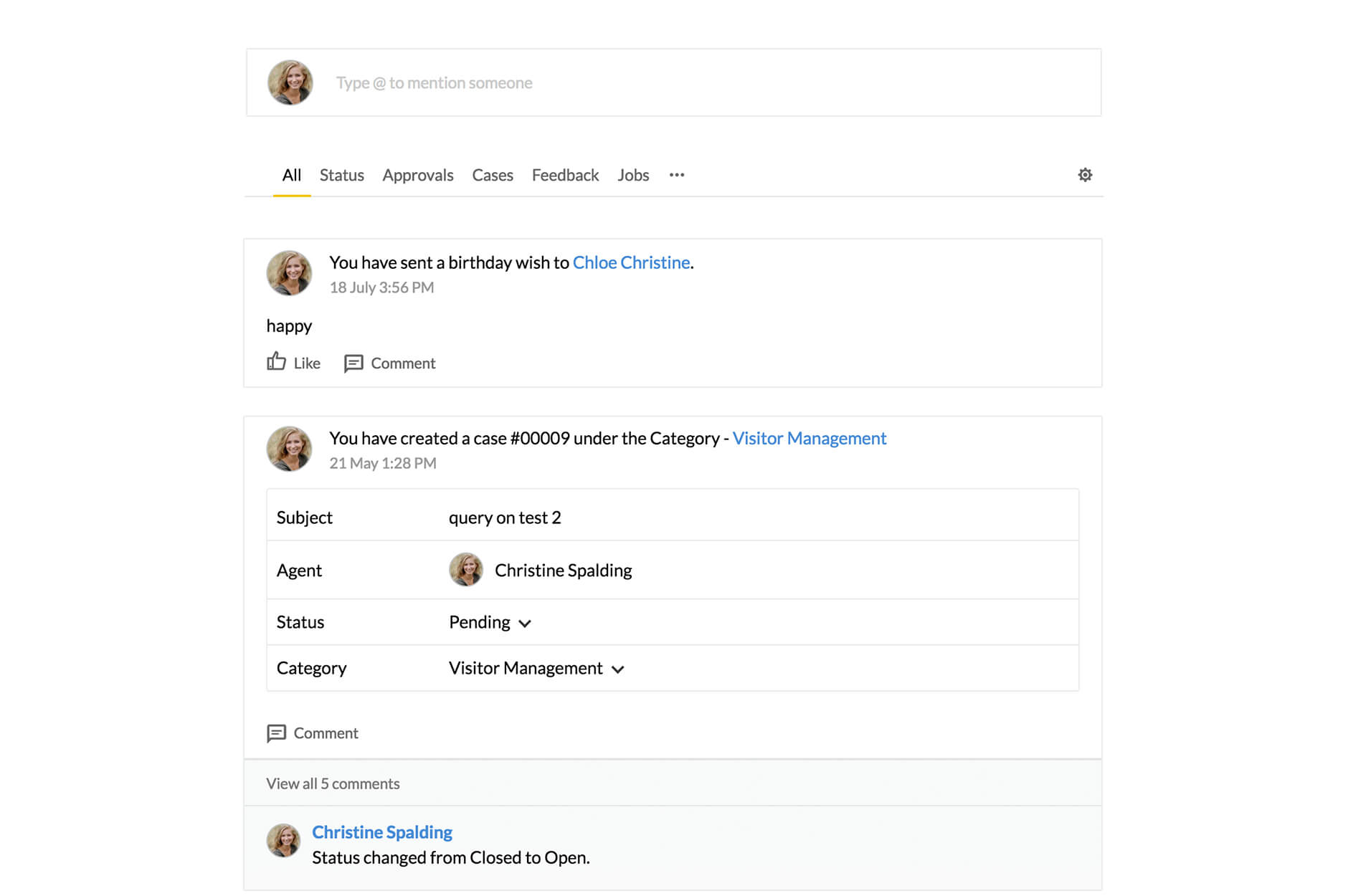The screenshot displays a Facebook interface with the main focus on a particular post and sections related to administrative tasks. At the top of the page, there is a search bar that reads "Type @ to mention someone." Below this, there is a profile picture of a woman with blonde hair. Next to the profile picture, a birthday wish has been sent to Chloe Christine with just the word "Happy" and a timestamp reading "Sent 18th of July, 3:56 pm." There are also "Like" and "Comment" buttons underneath the birthday wish.

Above this post, several sections are visible, labeled "All Status," "Approvals," "Cases," "Feedback," and "Jobs," with the section "All" currently selected. Scrolling further down, a case has been created with the number 00009 under the category "Visitor Management." The case includes a notation about a particular post with the subject "Query on Test Two." The agent handling this is Christine Spaulding, and the status of the case is "Pending Visitor Management." This section appears to be part of an administrative or moderation panel used to manage and review user posts and interactions.